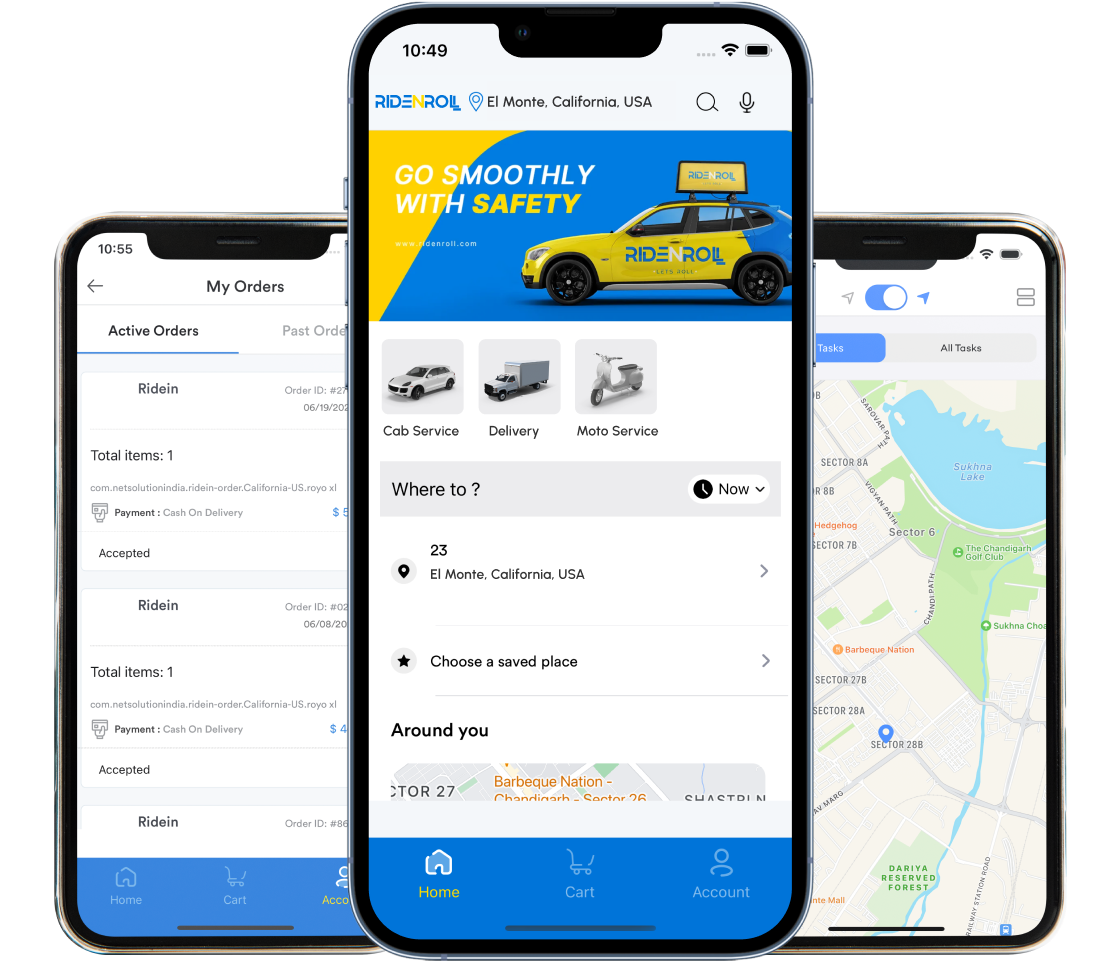In the image, three cell phones are displayed side by side, showcasing different screens of an app interface. 

The first cell phone on the far left displays an order tracking screen. At the top, it reads "My Orders" followed by a section titled "Active Orders." Below this, details of an ongoing order are shown: product name "R-I-D-E-I-N," a total of 1 item, with payment method listed as "Cash on Delivery." The order status is noted as "Accepted." Further down, it restates "Ride In" and confirms 1 total item.

The middle cell phone screen is larger and shows the time as 10:49. It features an image of a blue and yellow vehicle with the label "Ride Roll" (spelled out as R-I-D-E-R-O-L-L). Below this vehicle image are multiple service options: "Cab Service," "Delivery," and "Moto Service." The screen also has input fields for "Where To" and "Almonte, California, USA," along with a prompt to "Choose a Saved Place."

The third cell phone on the far right displays a map. The map includes a blue area representing a lake, surrounded by green areas denoting land or grassy regions. Several landmarks are marked, using orange and green text to differentiate them.

Overall, the image captures different functional aspects of a multi-service mobile application from order tracking and service selection to geographic navigation.